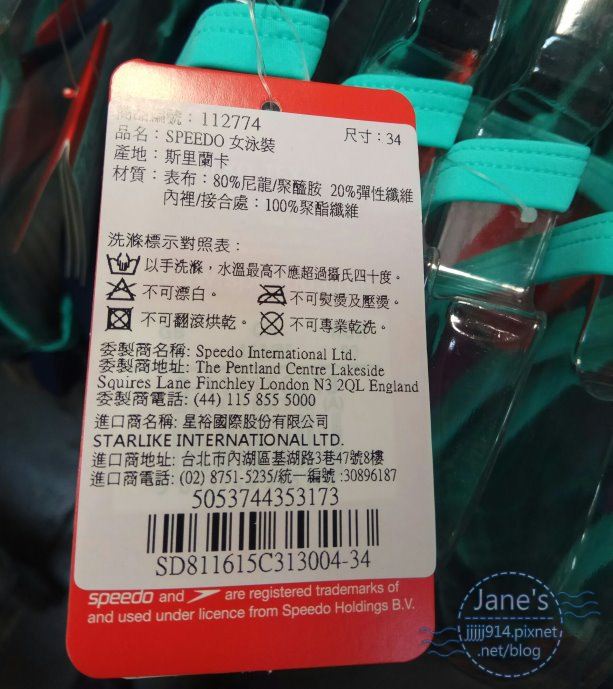The image depicts a close-up of a red clothing tag adorned with a white sticker featuring multiple lines of text. At the top of the sticker, in bold flesh-colored letters, the number "112774" is prominently displayed. Directly beneath this number, the brand name "Speedo" is written, with the majority of the surrounding text in Chinese characters. Towards the bottom of the sticker, there is a barcode, below which it states in English that "Speedo and the Speedo logo are registered trademarks of and used under license from Speedo Holdings BV." Supporting this description, there is a teal-colored strap behind the tag, suggesting it may be attached to an item of swimwear or athletic clothing. In the bottom right corner of the image, a circle watermark contains the text "James JJ JJ J 914.pics net.net/blog," indicating the source of the photograph.